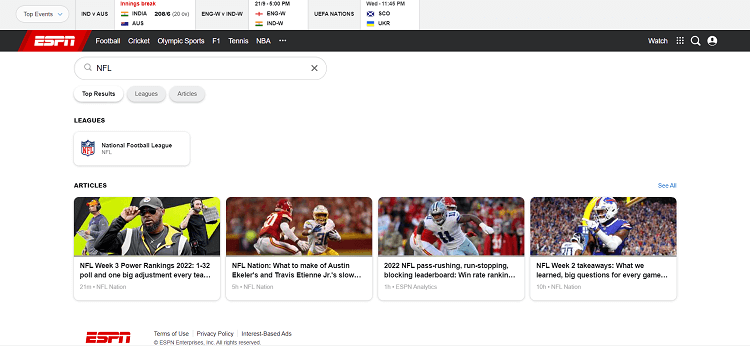This is a screenshot of the ESPN homepage, meticulously detailed with various sections and elements. The top edge of the page has a gradient color that transitions from light blue to light gray. The page is divided with the upper half featuring a black background and the lower half in white. 

In the top left corner, there is a white tab labeled "Top Events" in black font. Adjacent to this tab, separated by a vertical line, is an entry marked "IND vs AUS" with another line indicating a break in innings, and the teams India and Australia listed below with their respective flags. Next to it, another white space shows the match "ENG-W vs IND-W" along with the time "21:9 5 p.m." displaying the two teams beneath it. Farther right, within the same bar, is the "UEFA Nations" section indicating a time for the match "SCO vs UKR" also detailed with their flags.

Moving towards the right side of the black border, there's a prominent red rectangle inscribed with "ESPN." Next to it, are six sports listed in white, followed by an ellipsis and the word "Watch" on the far right. Below this, there are three dots forming a square, followed by white icons for search and profile.

Beneath this top section, a highlighted search bar reads "NFL," accompanied by a white tab labeled "Top Results" and two gray tabs for "Language" and "Articles." On the left-hand side, in bold black font, the word "Leagues" appears, followed below by "National Football League." The section continues with a list of articles, each accompanied by a football image and two lines of descriptive text beneath each thumbnail.